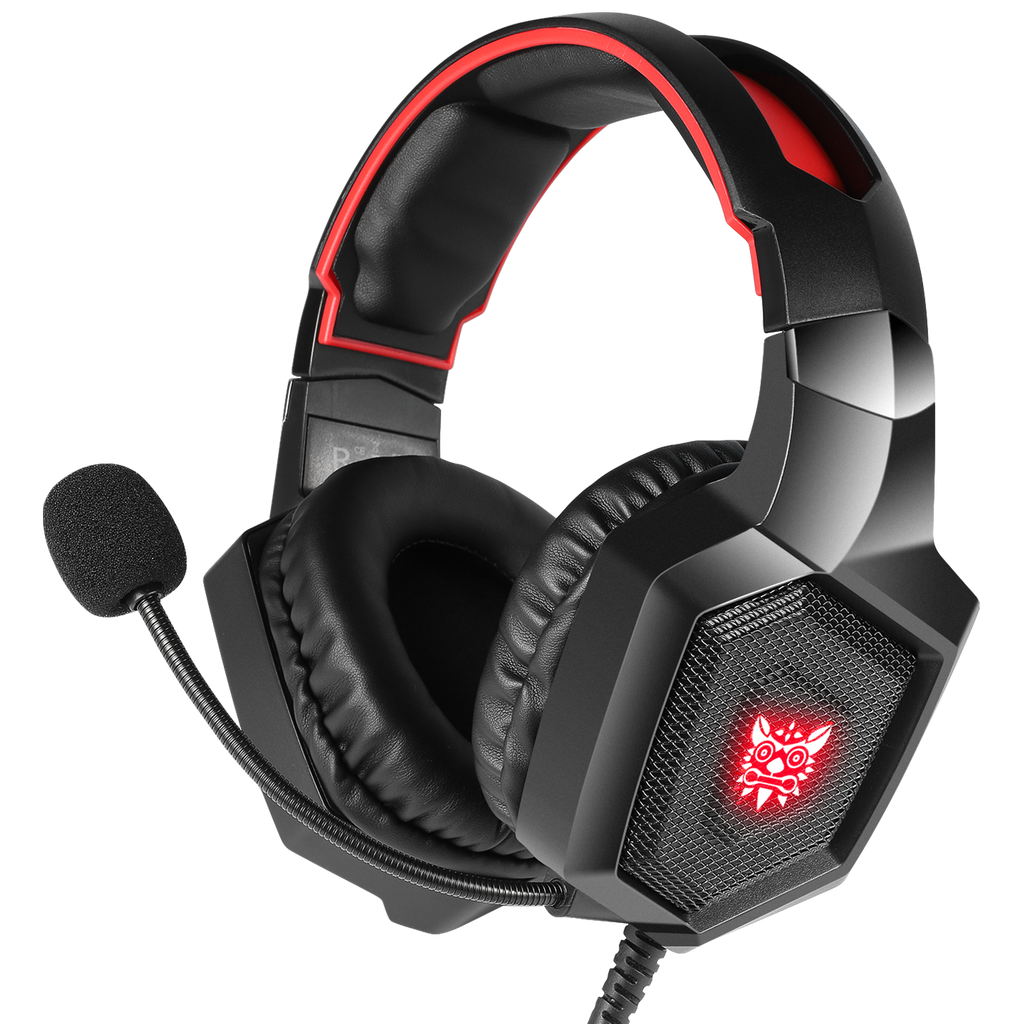The image shows a detailed, close-up view of a gaming headset. The headphones are primarily black with red trim along the top cushion, and they feature black pleather earpads for comfort. The outer flat surface of the ear sections has a hexagonal shape with a black mesh lining. Prominently displayed on each side is a glowing red and white logo depicting a dragon's face, reminiscent of ancient Japanese artwork. The headset is wired, with the connecting wire visible at the bottom, though it's cut off in the image. Attached to the headphones is an adjustable microphone with a black, fuzzy tip. The overall image is well-lit and clear, set against a white background.